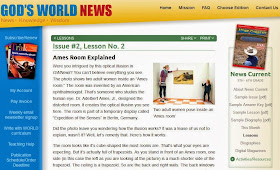The image depicts a webpage titled "God's World News," prominently displayed in the upper left corner. The phrase "God's World" is written in blue, while "News" is in red. Below this title, in faint red font, there is text that appears to start with the letter "W," though its exact content is unclear due to the poor resolution of the image. 

On the right side of the page, there is a horizontal navigation bar located centrally, featuring tabs that likely read: Home, Mission, FAQs, and Contact Us, with "Contact Us" being the last option on the far right. Beneath this navigation bar, a yellow section runs across the page, slanting lower on the left than on the right.

To the left of the page, a vertical blue navigation menu contains six items written in white font. Adjacent to this menu is a photograph resembling the cover of a magazine, followed by a section that appears to start with "I don't know my..." and "pay something," though the text is not entirely clear.

In the center of the page, a thin green strip displays text in white font. Below this green strip is a segment reading "Issue Number 2, Lesson Number 2" and "Ames Rome Explained."